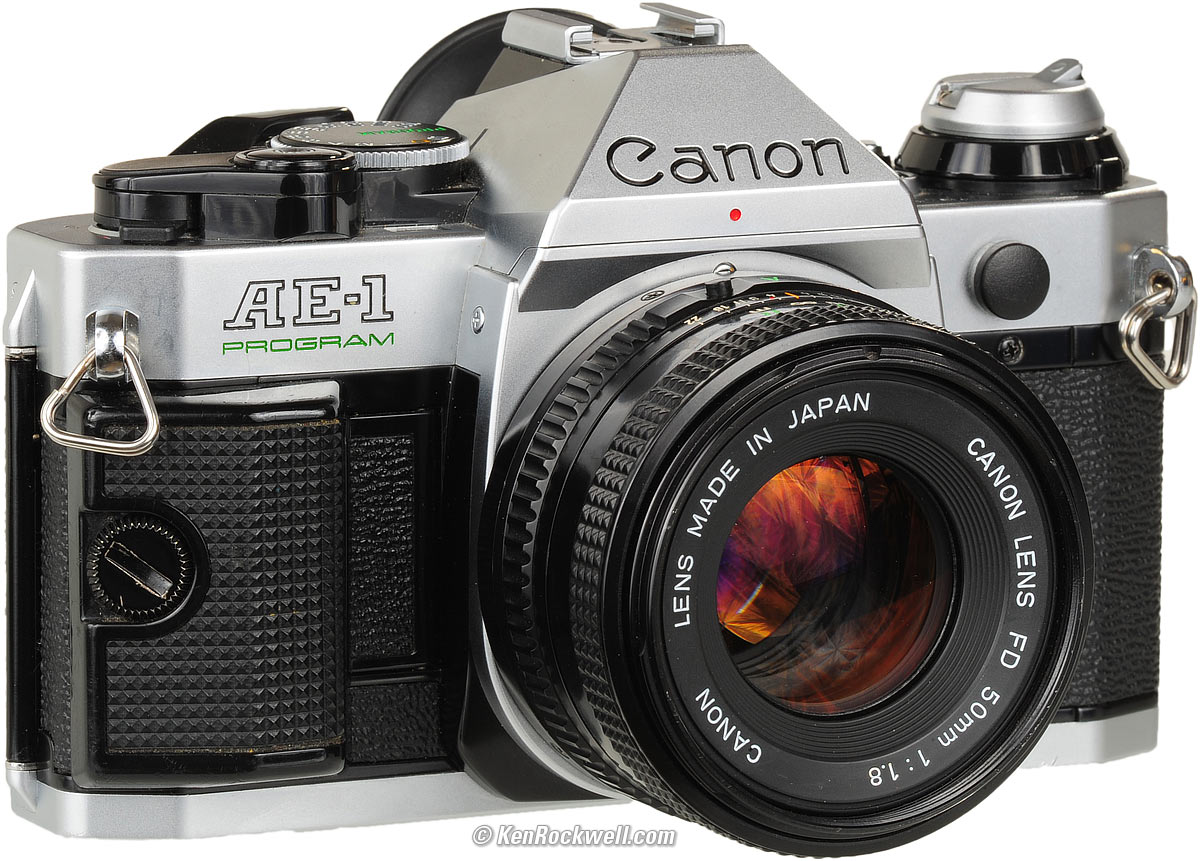The image depicts a Canon AE-1 Program camera characterized by its two-tone design, with a sleek silver top and a contrasting black bottom. The camera features black plastic side pieces for added grip. Its lens, prominently facing the viewer, has an orange tint caused by the reflection of light. Surrounding the lens, which is black around the edges, is white capitalized text that reads: "Lens Made in Japan, Canon Lens FD 50mm 1:1.8, Canon." The top center of the camera bears the iconic "Canon" logo, while the left side is marked with "AE-1" followed by the word "Program" in green letters. Additionally, there are two metal clips on either side of the camera designed for attaching a shoulder strap.